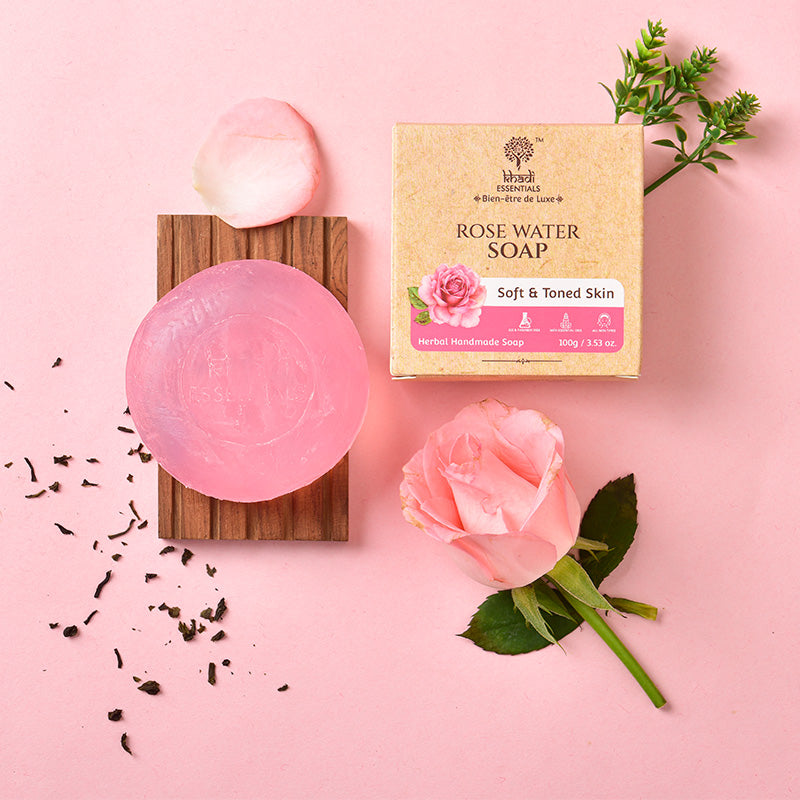The image features a soft gradient pink to white background. On the left, a round, pink glycerin soap rests on a wooden soap holder, adorned with a single rose petal on its upper edge. To the right, a beige box with brown lettering reads "Kadi Essentials Bien-Etre Deluxe Rose Water Soap." The box, embellished with an image of a pink cabbage rose, promotes "Soft and Toned Skin" and "Herbal Handmade Soap." Below the box lies a pink rose with a green stem and leaves, with additional green leaves visible at the top right of the box. The soap appears transparent and slightly pink, resembling glycerin.